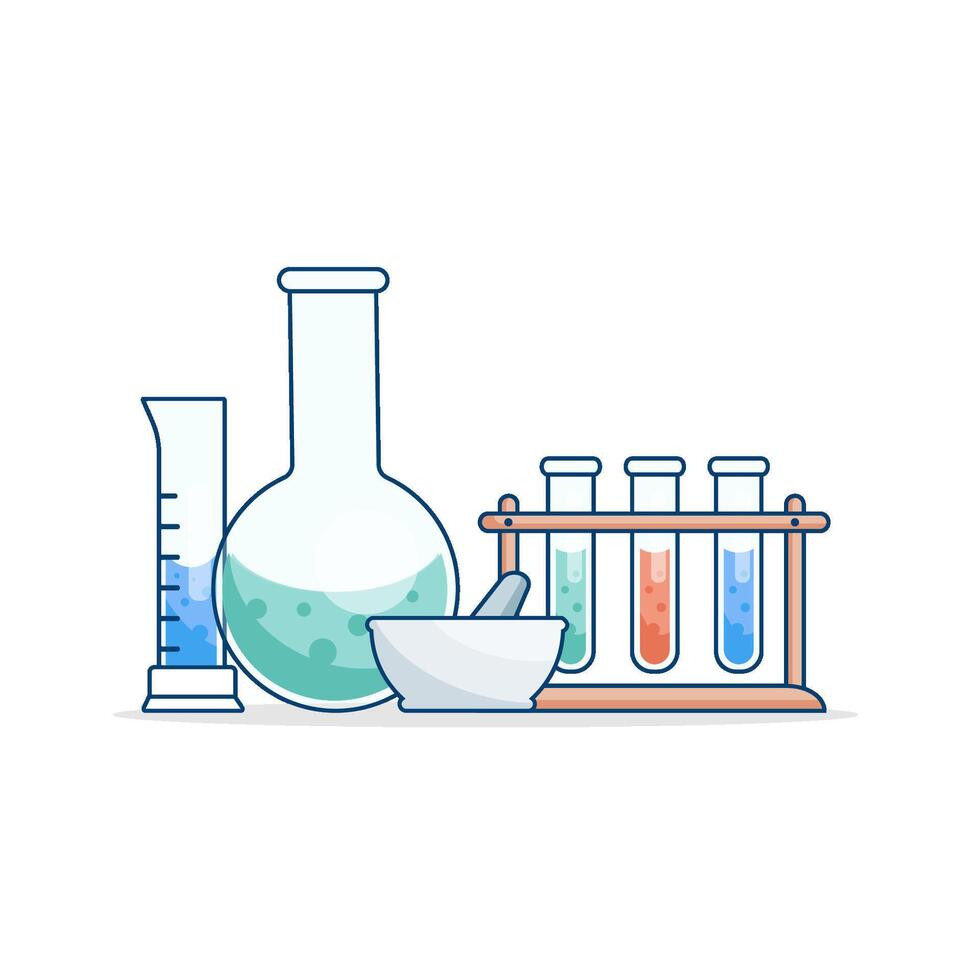The image is a simple, animated clip art illustration of a chemical set typically seen in a science class. Set against a white background with no border or text, the scene features various laboratory glassware. On the right side, there is a wooden test tube rack with a horizontal rod and two vertical supports at each end. It holds three test tubes: the one on the right contains a blue liquid filled halfway, the middle one contains an orange liquid, and the left one contains a green liquid. Next to the test tube rack is a round-bottom flask, about half full with a green substance and topped with a long tube. To the left of the flask is a tall, cylindrical beaker with black horizontal markings, filled to the fourth mark with a blue liquid. The overall style of the illustration is rudimentary, with even black line art defining the white-outlined shapes, giving it a straightforward, almost clip-art appearance.